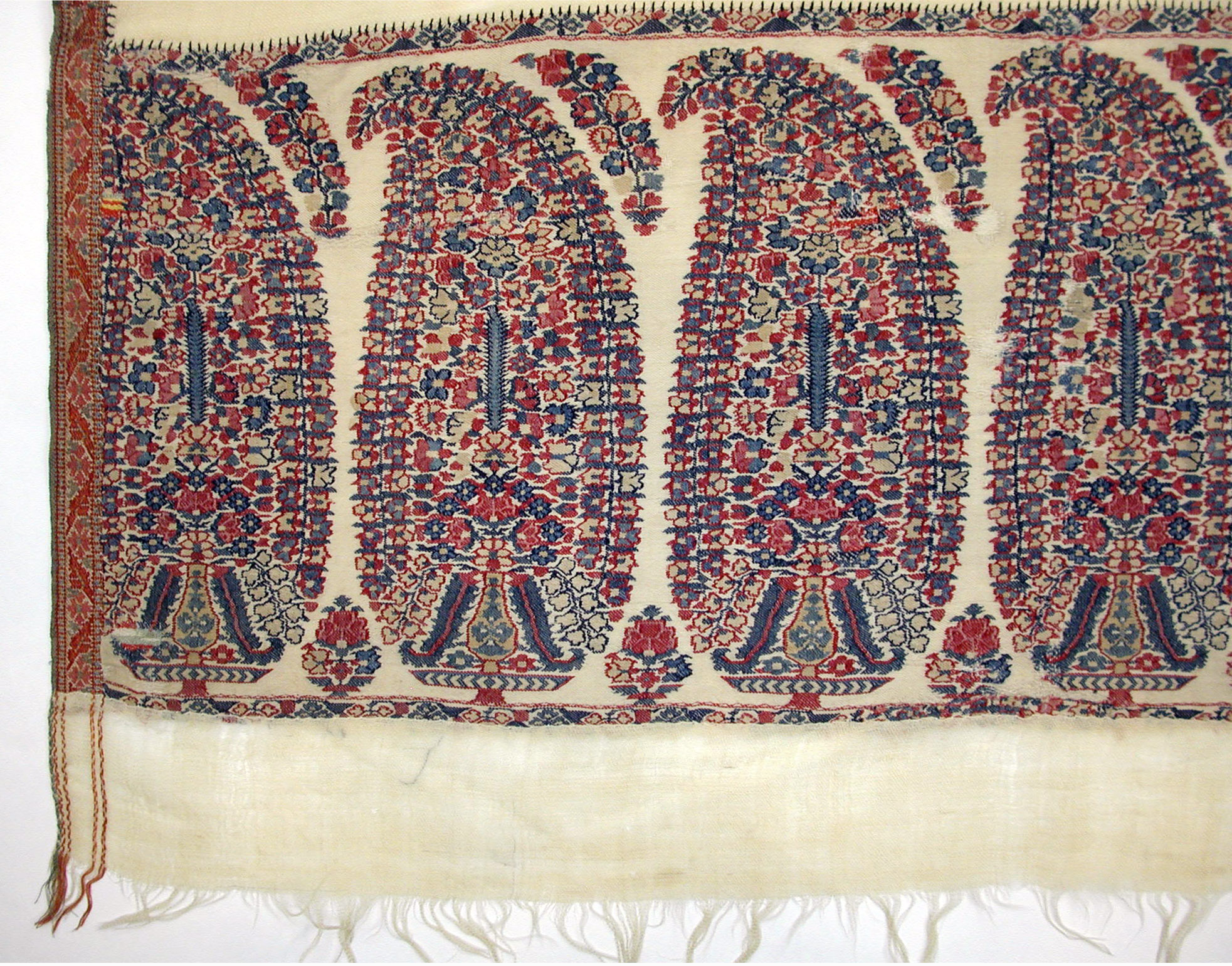This image showcases a thin, cream-colored tapestry that is intricately designed with an array of vibrant reds and blues. The central design features four identical teardrop patterns adorned with floral motifs. These teardrop shapes are positioned symmetrically, creating a rhythmic and balanced appearance. Each pattern contains swirling ovals and upward-curving flowers on the right-hand side, adding a fluid motion to the composition. Additional flowers anchor the bottom right of each teardrop, while leafy shapes intersperse the designs, enhancing the textured floral theme. The tapestry is bordered all around and features noticeable fraying at the bottom, with cream-colored strands extending from the edge, signifying its age and delicate nature. The overall imagery evokes the essence of a powerful, decorative piece, rich in color and intricate details.